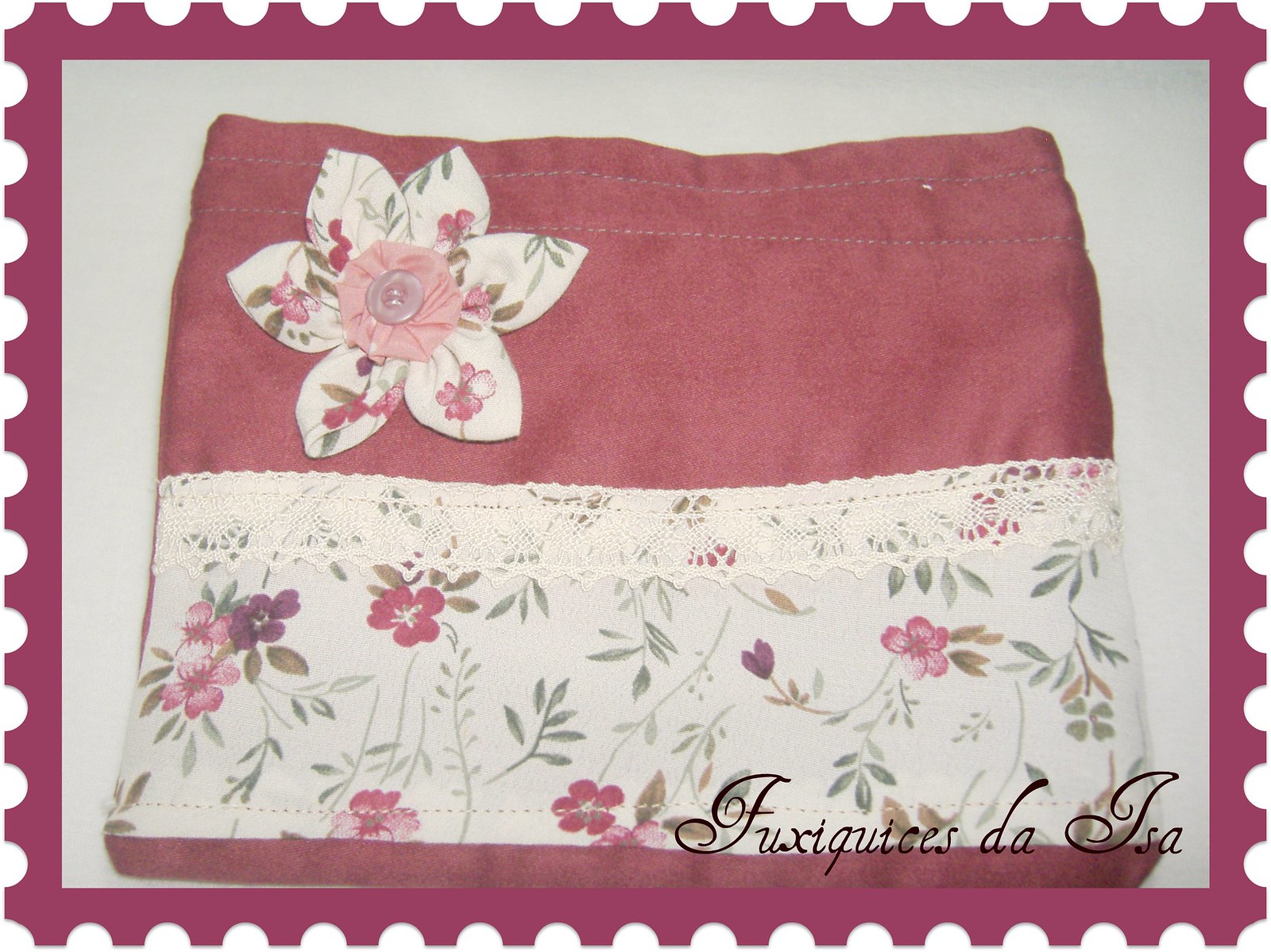This close-up image appears to feature an elaborately sewn square-shaped fabric piece framed by a dark pink, postage stamp-like border with a gray background. The upper portion of this fabric showcases a flower with multi-colored petals, having a tan background and pink hues. The center of this flower is accentuated with a light pink circle and a clear button. Below the flower, there's a skirt-like design made from the same material as the flower's leaves, adorned with lace on the upper edge. The bottom portion reveals a sliver of dark pink fabric. Across the bottom of the image, there is black cursive lettering that appears to be in another language, possibly reading "FUXIQUICESDAISA."